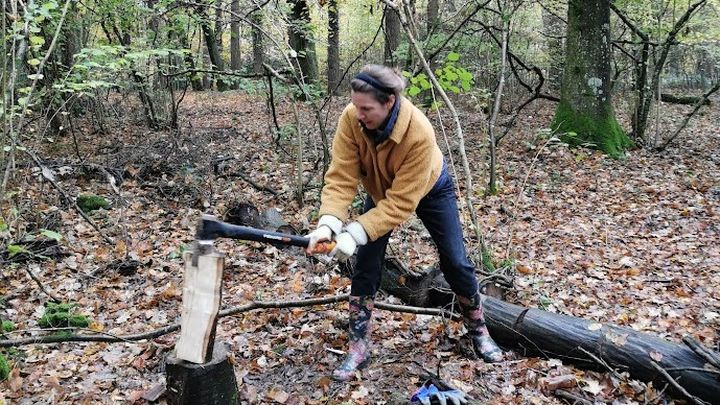In this detailed photo set in a forested area, a Caucasian woman, possibly in her mid-30s, is captured mid-action as she chops wood. The ground around her is a carpet of brown and light brown fallen leaves, suggesting it is either fall or winter. She stands in the center of the image, slightly leaning forward and to the left, focusing intently on a block of wood she is cutting with a black-handled axe. The wood is positioned on a tree stump, and her axe has just begun to penetrate the top of the log. She wears a blue shirt layered under an orange jacket, blue jeans, and flower-patterned rain boots. Her brown hair is neatly pulled back and secured with a blue headband, and she has white gloves with orange-tipped fingers on her hands. In the backdrop, slender green-leaved trees line the scene from left to right. Some notable features include three black branches rising from the ground on the right side of the image, and a round tree with green moss at its base to the left. Behind her left foot lies a fallen tree trunk, stretching out of view. The woman’s determined stance and the scattered leaves accentuate the serene yet industrious atmosphere of the forest setting.